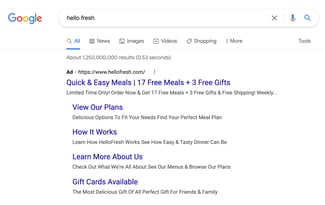This image is a close-up screenshot of a computer screen displaying the Google search results page. Dominating the upper left of the image is the iconic Google logo, followed by the minimalistic Google search bar. Within the search bar, the term "Hello Fresh" is typed, indicating a query for information about the meal delivery service. Below the search bar, the top result is marked as an advertisement ("ad") for Hello Fresh, with the URL "https://www.hellofresh.com" clearly visible. 

The main headline of the ad is prominently displayed in clickable blue text, proclaiming "Quick and Easy Meals, 17 Free Meals and 3 Free Gifts." Beneath this headline are four secondary links, also in blue, each offering additional navigational options for the user: "View Our Plans," "How It Works," "Learn More About Us," and "Gift Cards Available." 

Accompanying each blue link, as well as the main headline, are brief descriptions in black text, although the contents of these sentences remain unreadable due to the small size of the screenshot. The overall layout is typical of Google’s structured ad presentation, aimed at providing easy access to an array of services offered by Hello Fresh.